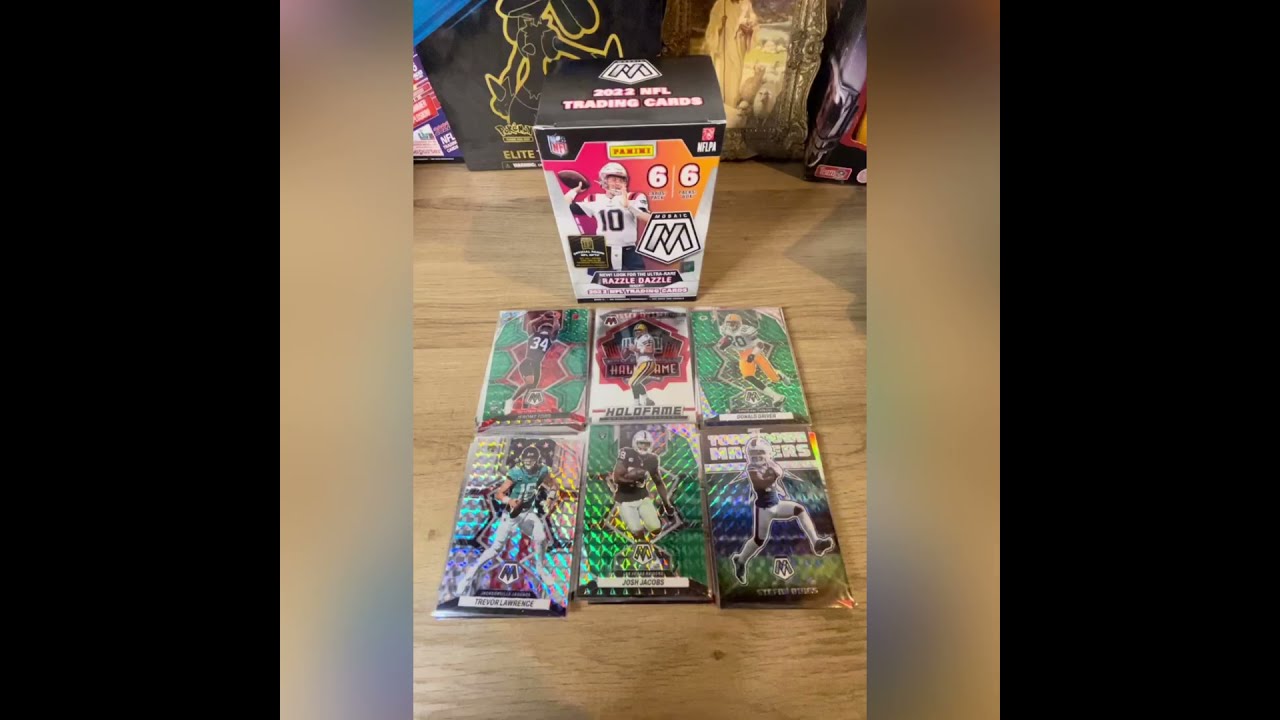This detailed color photograph features a display of 2022 NFL trading cards. The image is bordered by vertical black bars on the left and right, each about an inch and a half wide. Nestled inside these black borders, there are gradient bands in shades of gold, beige, and blue, fading into each other. The central photograph showcases a collection of six holographic football trading cards arranged in two rows of three, laid out on a medium-colored wood floor. These appear to be specialty cards, likely taken from the prominently displayed box behind them. The box, marked "2022 NFL trading cards," features an image of a football player wearing a number 10 jersey, depicted in a white outfit and holding a football. The bottom of the box displays the phrase "Razzle Razzle," and it includes color elements of black, white, red, pink, and orange. Additional products are visible in the background, though they are partially cut off and less discernible.